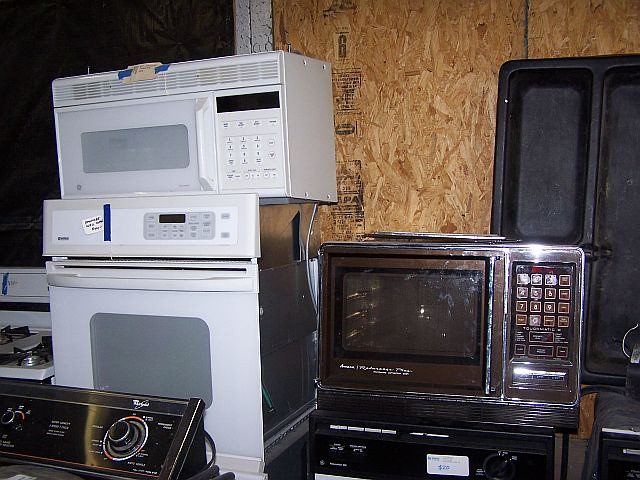This photograph features a collection of vintage kitchen appliances, all stacked haphazardly against a wooden wall. Dominating the lower left corner is an aged white stove with two visible burner tops, each covered with dark metal grates. This stove carries a noticeable strip of blue tape and possibly a note, though the writing is indistinguishable. Right beside it sits another white oven with gray buttons lining its right side and a similar blue tape strip affixed to it. 

On top of this oven rests a white microwave, discernible by its gray glass door and blue tape marking. Adjacent to this stack, there's a retro brown microwave with large, distinctive square buttons and a dark brown, see-through glass door, perched atop another unspecified electronic device. Throughout the assortment, the appliances display a range of wear including scratches and dents, enhancing their nostalgic appearance with a well-used, battered charm. The overall scene faces outward at a diagonal angle, adding to the chaotic yet intriguing composition of these bygone-era kitchen essentials.